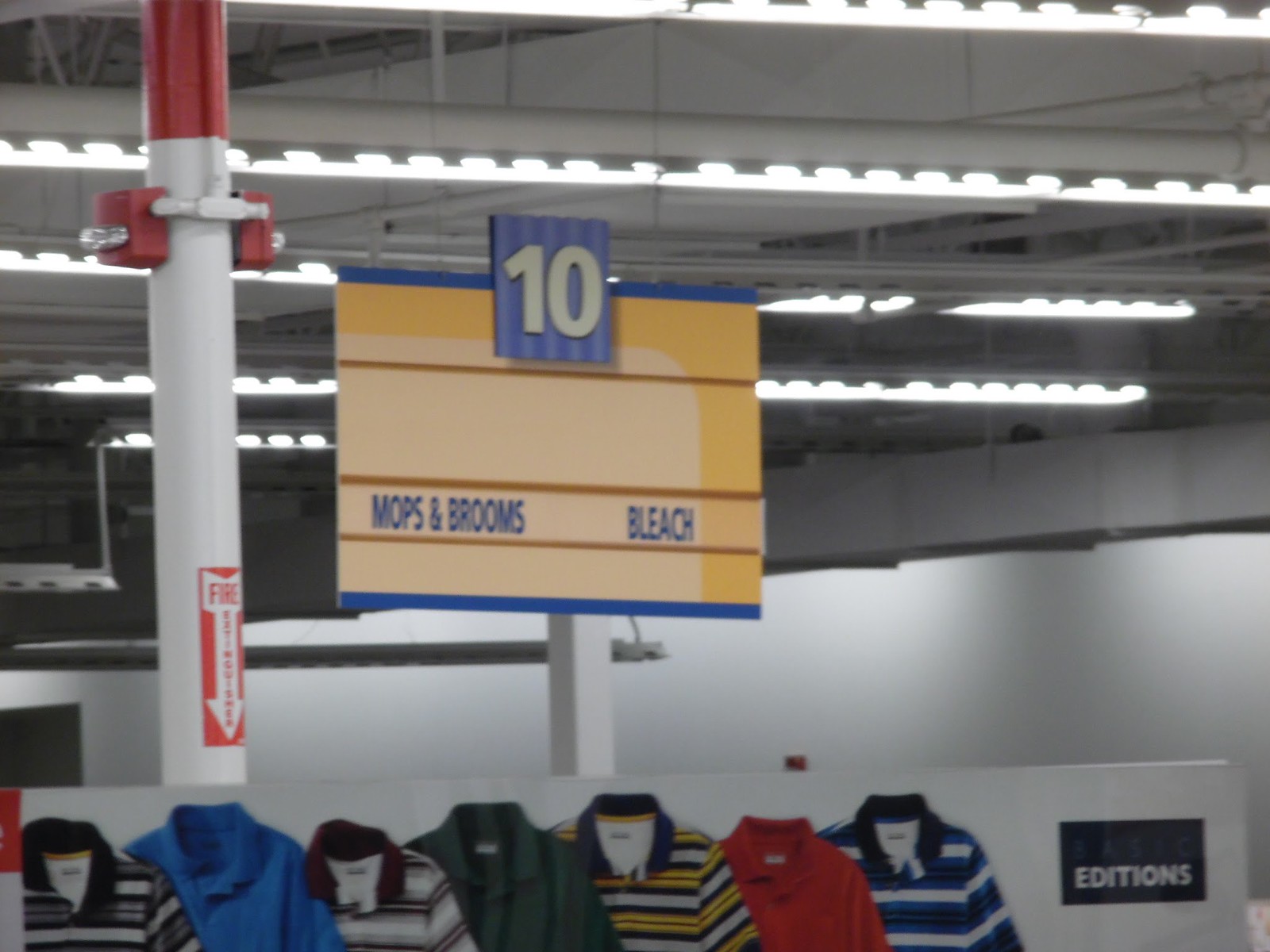This image, taken inside a store, features a prominently displayed aisle sign hanging from the ceiling in aisle 10. The background of the sign is a combination of yellow and light blue stripes, with the number "10" in white lettering. Below, in blue letters, the sign indicates "mops and brooms" alongside "bleach." The ceiling, adorned with large rectangular shapes, supports suspended oval-shaped fluorescent lights emanating a white glow. A significant white structural pole, enhanced with a red arrow label for a fire extinguisher and accompanied by two fire alarms, stands to the left of the aisle sign. Below the sign is a white wall exhibiting a selection of men's collared polo shirts in various colors and patterns, including striped blue, green, and yellow, as well as solid blue.